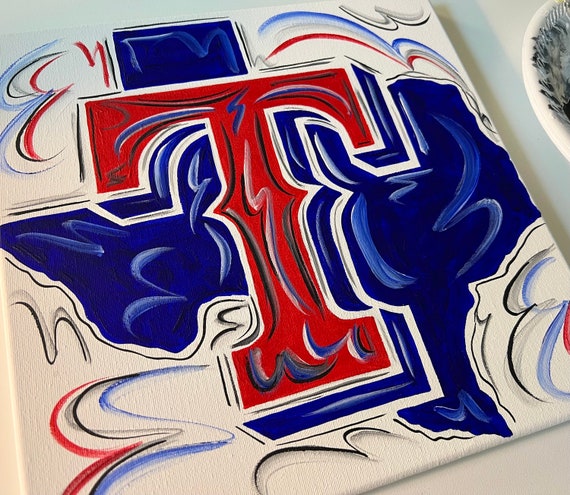The image features a detailed painting on a white canvas that rests atop a white surface. The centerpiece of the painting is a large, uppercase red letter "T," rendered in a hand-drawn serif font with two prominent bulging spikes emanating from the center of the downstroke. This "T" is adorned with intricate black, blue, and white swirls.

Behind the "T" is the outline of the state of Texas, painted in a deep royal blue. Further enhancing the composition, each of the four corners of the canvas is decorated with additional swirling designs in red, blue, and black, mirroring the patterns found within the "T." 

In the upper right-hand corner of the image, there's a glimpse of a white bowl with a blue design on the inside, along with the visible shadow cast by this setup, adding a subtle depth to the overall depiction. The clean wrapping of the white canvas around its frame suggests the use of oil paint, giving the artwork a polished and textured appearance.